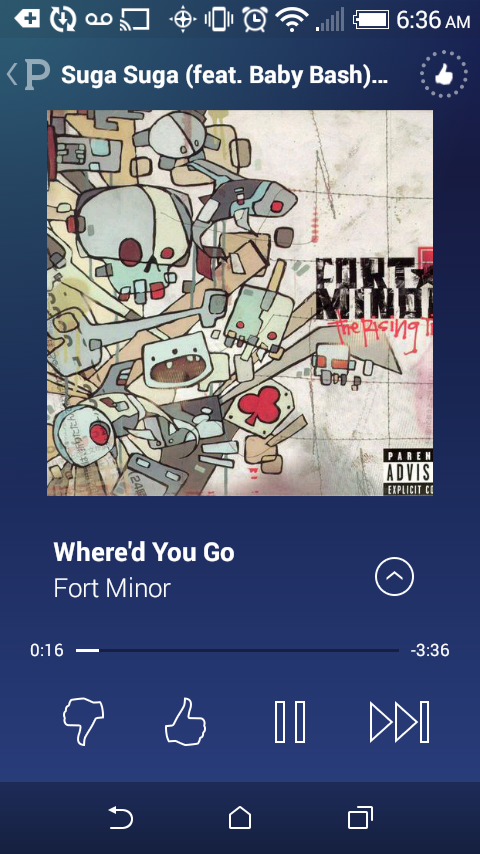This detailed caption integrates and refines the different elements described across the three captions:

This is a full-color digital screenshot of a mobile music player taken at 6:36 AM with a fully charged battery and one bar of signal. The screen displays various status symbols including an alarm icon and settings like a house, swooping arrow, and multiple boxes at the bottom. The music player's interface shows the song "Where'd You Go" by Fort Minor, 16 seconds into the track with 3 minutes and 36 seconds remaining. The album cover, centered in the image, depicts a stream of skulls and humanoid figurines flowing from left to right, with the band's name, Fort Minor, partially obscured but identifiable, written in black. Below, the album title "The Rising Tied" is printed in red font. A parental advisory label for explicit content appears prominently in the bottom right corner. Control options including thumbs up, thumbs down, pause, and fast forward are located near the bottom of the screen.